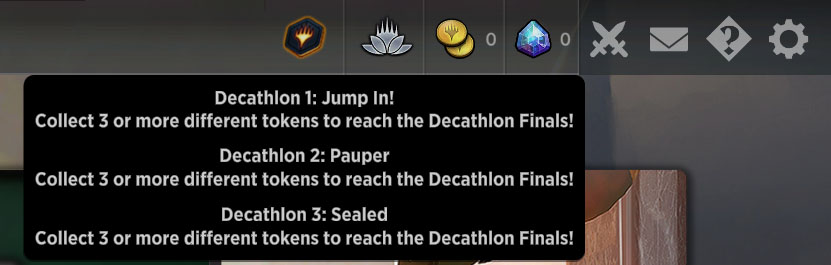The image is a rectangular screenshot from a mobile game app featuring a gray background. Prominently displayed is a black, rectangular text box situated in the bottom left quadrant of the image, which features white instructional text. The text outlines three game challenges: "Decathlon1: Jump In, collect three or more different tokens to reach the Decathlon Finals." "Decathlon2: Popper, collect three or more different tokens to reach the Decathlon Finals." "Decathlon3: Sealed, collect three or more different tokens to reach the Decathlon Finals."

In addition to the text box, there is a stained wood door frame partially visible on the right side of the image. At the top of the screen, a gray border houses several small icons that are part of the game interface. These icons include a gear, question mark, envelope, crossed swords, a blue gem, gold coins, a flower, and an octagon with a flame in the middle, indicating various game elements and functions.